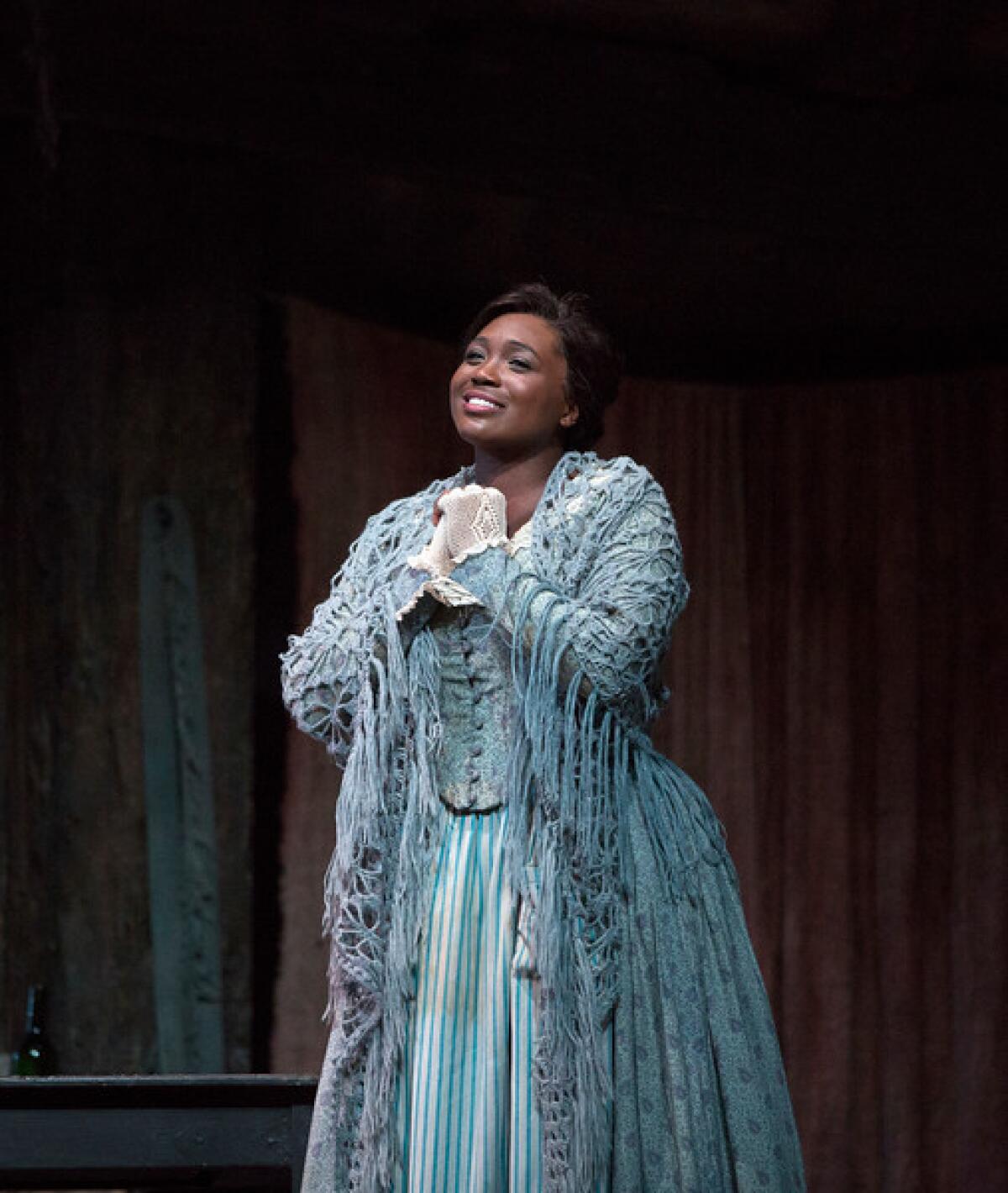The image depicts a woman standing on a stage, framed against a backdrop of dark brown curtains with additional white, blue, and grey curtains on the left side. She has short brown hair and a warm, slightly smiling expression with her teeth visible. The woman is wearing a long, blue vertically striped dress paired with a blue vest adorned with many buttons. Over her outfit, she drapes a blue crocheted shawl or cap, and she holds a white crocheted handkerchief in her hands. The dress and shawl feature intricate, net-like patterns that are semi-transparent in some areas. She complements her attire with white gloves, adding to the formality of her appearance. The overall setting suggests that she is participating in a play or a performance, conveying a sense of confidence as she faces the audience.